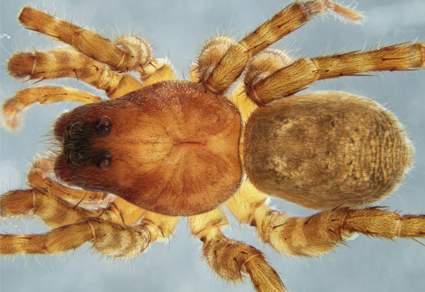This detailed close-up photo (possibly a realistic painting) of a tarantula reveals intricate details of its anatomy against a plain gradient background. The tarantula, occupying about 90% of the centered frame, is predominantly golden yellow with its abdomen or thorax showing a darkish brown, wool-like texture. The area around its multiple eyes—either six or eight small black dots—is a brighter orange. The spider’s eight legs are somewhat translucent, adorned with faded brown stripes, and covered in fine, fibrous hairs, giving them a corn stalk appearance. The legs and the furry abdomen enhance its creepy, realistic look. The tarantula has what appears to be two small, delicate pinchers (possibly mistaken for antennas) near its front, and its large, bulbous rear emphasizes its hairy, detailed structure. The background behind this menacing arachnid is a solid gray gradient with no other distractions, ensuring that the tarantula remains the sole focus of this unsettling yet fascinating image.